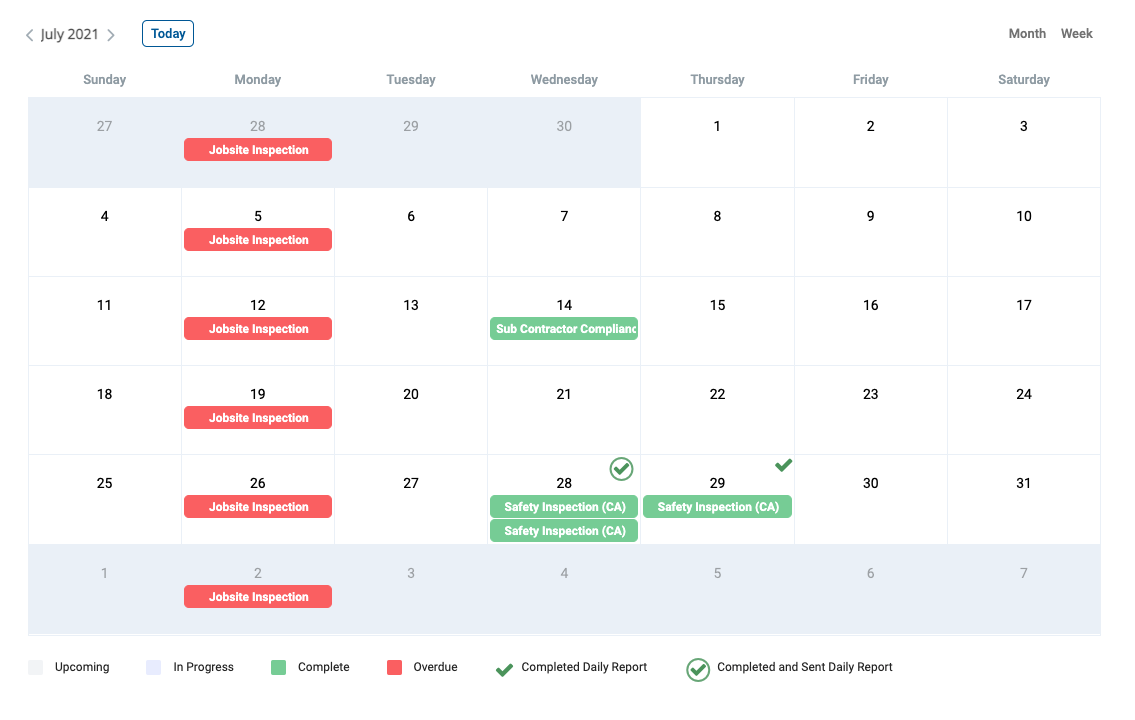A detailed image of a July 2021 calendar is displayed. The calendar features black text on a clean white background. The layout includes an overview of the month, the week, and the current day. The calendar starts by showing a couple of days from the end of the previous month, specifically from the 27th of June, and extends through the first week of August, ending on the 7th.

Within the calendar grid, all dates that do not belong to July are shaded in gray, contrasting against the standard black text used for the days within July. Each date from the 1st through the 31st of July is centered and displayed prominently in black text.

A pattern of red bars marks every Monday, suggesting significant, recurring events on these days. Additionally, there are several green bars and a few green logos scattered across the calendar, adding visual cues for specific dates. However, the exact details or meanings of these green logos are unclear as they are not easily legible.

The days of the week are written in a subtler gray text, providing a clear structure to navigate through the month. Overall, the design is tidy and functional, offering a straightforward view of the month of July with hints of upcoming activities in early August.